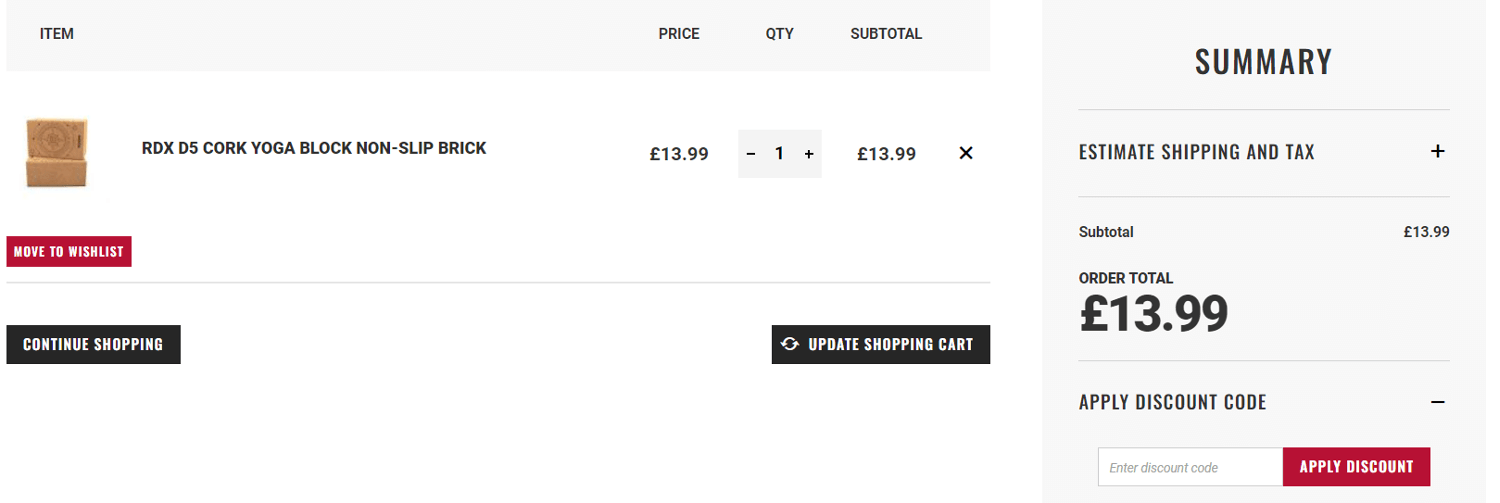Sure! Here is a more detailed and cleaned up caption:

---

The website features a two-column layout. On the left side, occupying about two-thirds of the width, there is an itemized list with headings that include "Item," "Price," "Quantity," and "Subtotal." Below this header, a boxed item is displayed but the visual details are unclear. The product, identified as "RDX D5 Cork Yoga Block Non-Slip Brick," appears to be a yoga accessory priced at £13.99. The quantity is set to one by default, with adjustable plus and minus buttons to modify the quantity. The subtotal for this item stands at £13.99. Beneath the product information, there is an option to "Move to Wish List."

Just below, a black rectangular button labeled "Continue Shopping" in white text invites users to continue browsing. Alternatively, users can update their shopping cart by selecting an option on the right side of the screen.

The right column, which is about a quarter of the page width, provides a summary section. This section allows users to estimate shipping and tax costs by clicking a plus button. The subtotal is reiterated as £13.99, matching the order total. There's also a prompt to apply a discount code; a field is provided for input, alongside an "Apply Discount" button for easy application.

---